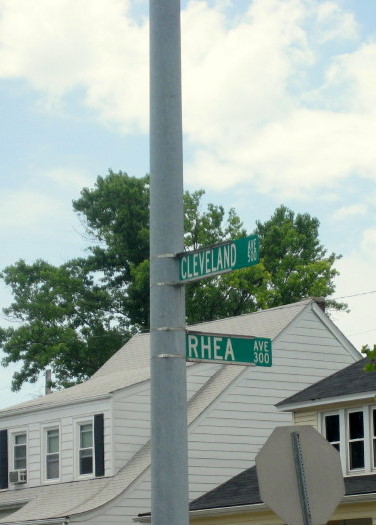This image captures a sunny street corner on a bright day with a striking blue sky adorned with fluffy clouds. The main focus is a street pole at the intersection of Cleveland and Ria, each indicated by green street signs with white font. Cleveland Avenue is at the top of the pole, while Ria Avenue signs horizontally below it, marking the 300 and 500 blocks respectively. Positioned at the lower right side is the back of a stop sign. The background features residential houses; one white with a beige roof, the other off-white with a black roof. Trees and power lines punctuate the scene, reflecting a typical suburban neighborhood, possibly located in the Midwest, South, or Northeast. The photo is taken from a low angle, as if standing at the foot of the pole, emphasizing the clarity of the street signs against the bright, clear sky.